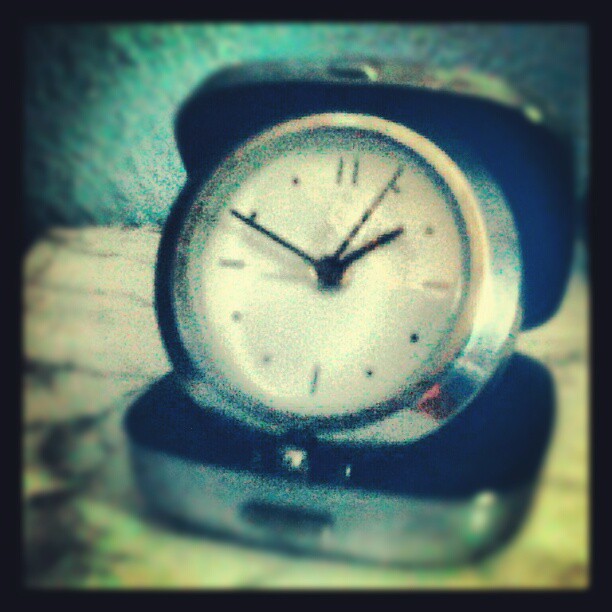The image presents a faded and blurry photo of a vintage-style alarm clock nestled inside an open, small silver briefcase. This retro clock, possibly dating back to the 1950s to 1980s, has a circular face with a pristine white background bearing black lines for seconds or minutes, and three black clock hands: two long and slender, and one short and wide. Despite the graininess of the picture, the clock shows a time of approximately 2 o'clock. The briefcase and clock rest on a light brown wooden table with noticeable darker grains running vertically. Behind the setup, a textured blue wall adds depth to the backdrop, contrasting with the smooth, silver frame of the clock and its case, embodying a harmonious blend of historical charm and functional design.